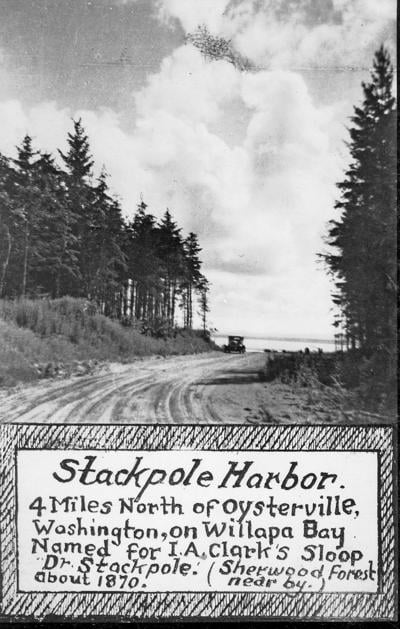This historical black-and-white photograph captures a wide, dirt road graced with numerous tire tracks, leading into the distance where an old-fashioned black box-like car, possibly a Model T, traverses the path. Flanking the road, tall grasses and vegetation give way to towering pine trees, their thick foliage climbing skyward. Above, a dark gray sky stretches out, punctuated by substantial, fluffy white clouds, hinting at daytime illumination. The barely discernible water in the background, as the caption clarifies, belongs to Stackpole Harbor, situated four miles north of Oysterville, Washington, on Willapa Bay—named in honor of I.A. Clarke's sloop, Dr. Stackpole. At the bottom of the image, a bordered rectangle features black diagonal lines framing a white rectangle that bears this informative caption. The caption also notes the nearby Sherwood Forest and dates the image to approximately 1870, emphasizing its vintage origin.